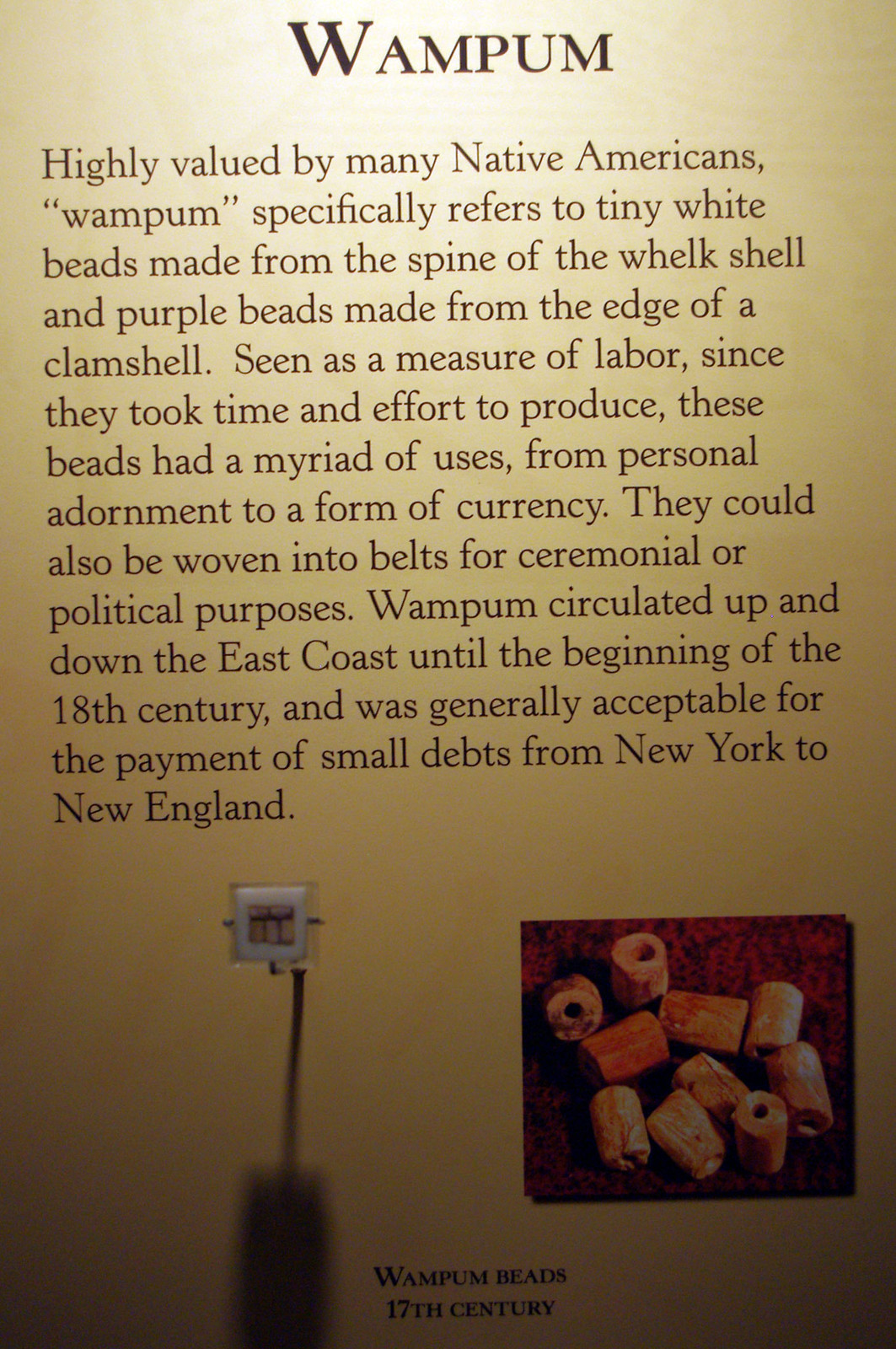The image depicts a museum display with informative text about Wampum, written in dark brown on a light tan background that is lighter at the top, possibly due to overhead lighting. At the top of the display, the title "Wampum" is prominently featured in large, bold black font. Beneath the title, the text reads: "Highly valued by many Native Americans, Wampum specifically refers to tiny white beads made from the spine of the whelk shell and purple beads made from the edge of a clam shell. Seen as a measure of labor since they took time and effort to produce, these beads had a myriad of uses, from personal adornment to a form of currency. They could also be woven into belts for ceremonial or political purposes. Wampum circulated up and down the East Coast until the beginning of the 18th century and was generally accepted for the payment of small debts from New York to New England." At the bottom right of the display, there is a picture of the wampum beads, with the caption "Wampum Beads 17th Century." Additionally, a white square is visible on the left side of the display.